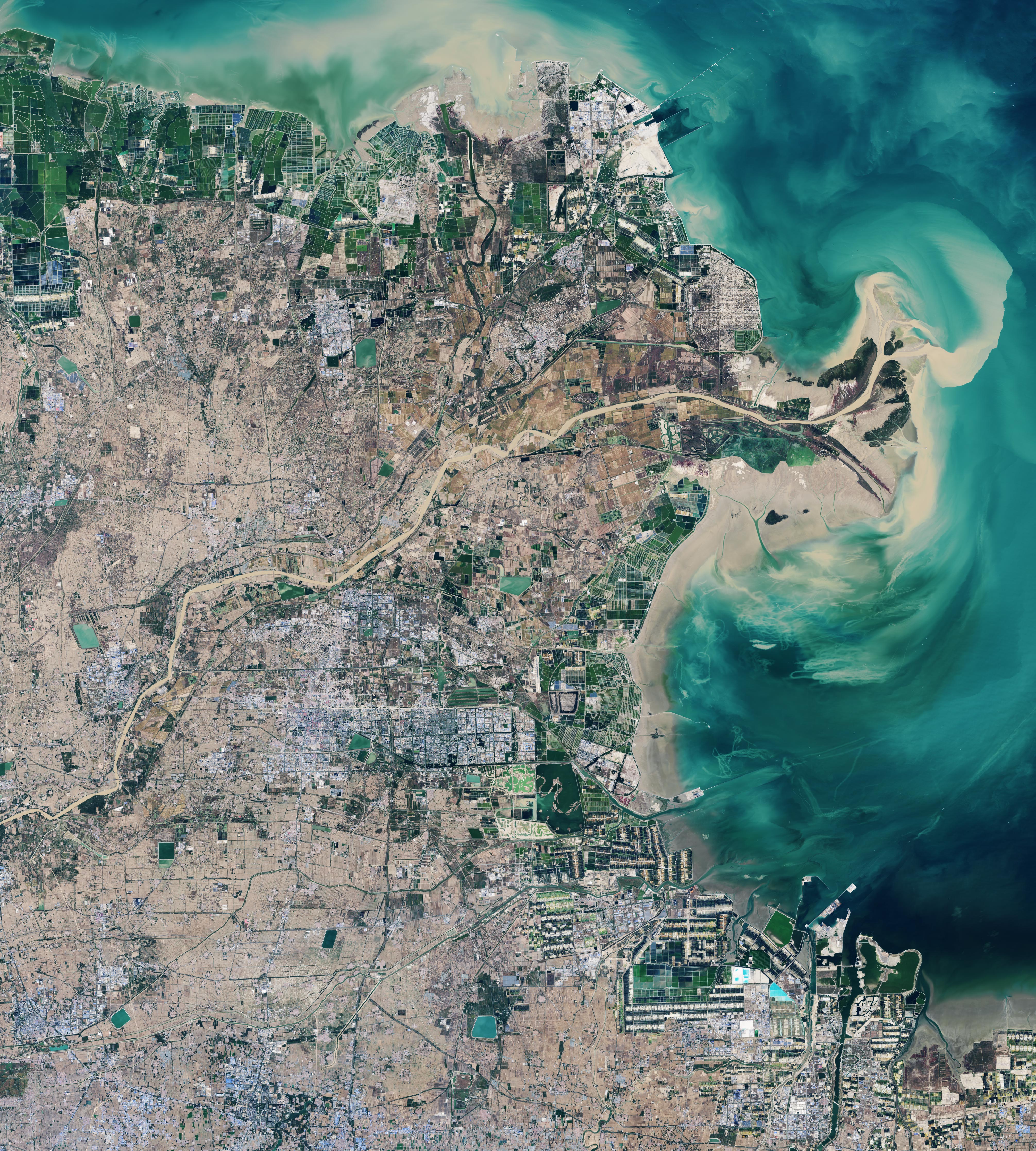This is an expansive aerial photograph, likely taken from an aircraft or a drone, capturing a coastline city next to a vast turquoise ocean. The aerial perspective offers a high-altitude view, similar to a map, showcasing the intricate details of the terrain below. The water along the coastline is a vibrant mix of dark blue and green, with flecks of aqua, giving it a tropical appearance. The coastline features a beach and diverse structures nestled in the brown earth, highlighting various buildings, houses, and possibly towns with differing population densities. A prominent road runs horizontally through the middle of the photograph, leading to the water's edge. To the upper left of the image, there is a significant patch of green fields, contrasting with the predominantly brown and dirt terrain. The scene is dotted with greenery, roads, and what appears to be a brown river winding through the land, offering a comprehensive and dynamic view of this coastal area.